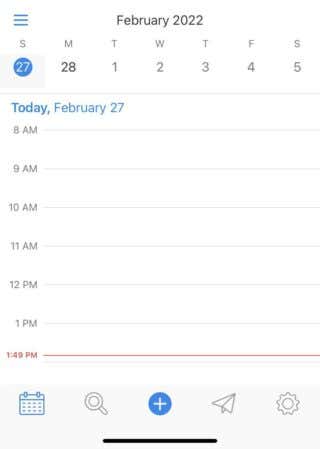This image features a digital calendar interface set for February 27, 2022. In the upper-left corner of the interface, three horizontal bars are stacked over one another, likely representing a menu. The date "February 22" is prominently displayed, followed by the first letter of each day of the week: S, M, T, W, T, F, S. Under "S" for Sunday, the date "27" is highlighted in white within a blue circle, while the date "28" is bolded. The numbers "1, 2, 3, 4, 5" follow in sequence towards the end of the week.

Beneath this row of dates, a gray line separates the top section from the hourly schedule. The current date "Today, February 27" is marked in blue text. The scheduled times are listed by the hour in black text, each separated by a gray line: "8 a.m.," "9 a.m.," "10 a.m.," "11 a.m.," "12 p.m.," and "1 p.m." At 1:49 p.m., a red line and “1:49 p.m.” text in red mark the current time.

At the bottom of the calendar, there is a light gray bar featuring several icons: a calendar icon in blue, a gray magnifying glass (likely representing search), a blue circle with a white plus symbol (likely for adding events), a paper airplane outlined in gray (possibly for sharing or sending), and a settings cogwheel outlined in gray.

Lastly, a black line horizontally bisects the interface at the bottom, adding to the clean, organized look.